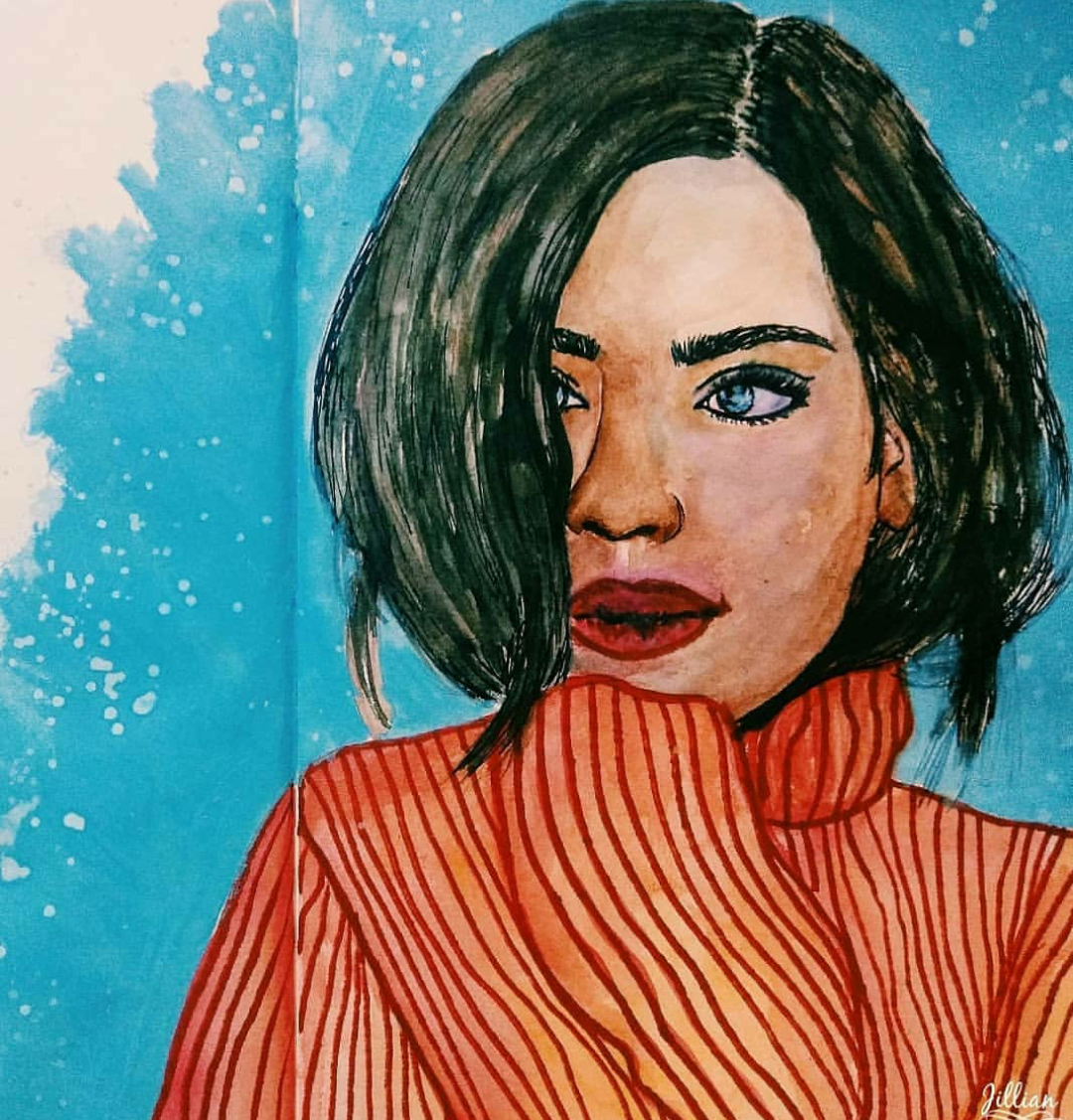This watercolor painting by Julian features a young, shy woman with striking blue eyes and dark black hair cut in a bob that falls just to her shoulders, partially covering her right eye. She wears a high-collared, over-length sleeved, orange turtleneck sweater with darker orange stripes. The woman's red lips are slightly parted, and her hidden hand is tucked under her chin as if in contemplation. The background is primarily a soft turquoise blue with white splotches and visible brush strokes, creating a serene and gentle atmosphere. The artist's beautiful calligraphy is signed in the bottom right-hand corner of the painting.